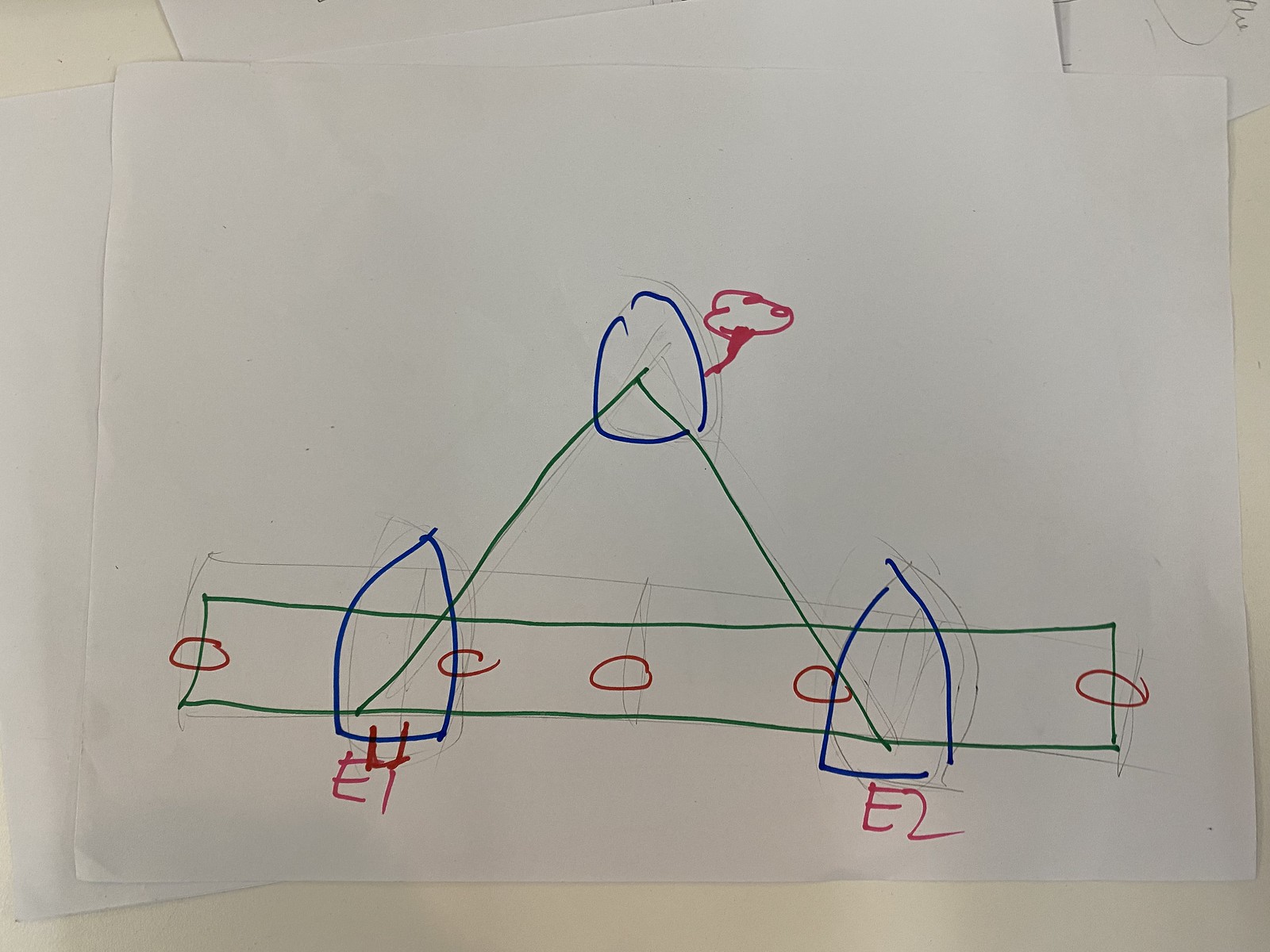This photograph showcases a line drawing executed in marker, meticulously centered on a rectangular piece of white paper. The main piece of paper rests atop another white sheet, which is slightly angled to the right, with yet another white sheet underneath, angled to the left, creating a layered effect. In the upper right corner of the composition, a smaller piece of white paper features what appears to be a sideways 'W' scrawled in pencil, adding an intriguing, almost cryptic element to the scene.

The central drawing is rendered in rich purple, green, and red hues. Dominating the center is a vivid red circle. From the circle emanates a triangular shape, at whose base lies a long, horizontal rectangle stretching across the lower side of the triangle. Flanking this rectangle on either side are two additional triangular shapes, creating a symmetrical, balanced aesthetic.

An enigmatic, red, swirling figure spirals from the top of the central red circle, lending a sense of dynamic motion to the otherwise geometric composition. Below the two bottom triangular shapes, the alphanumeric characters 'E4' and 'E2' are inscribed in striking red ink, possibly indicating some form of label or code, inviting viewers to ponder their significance.